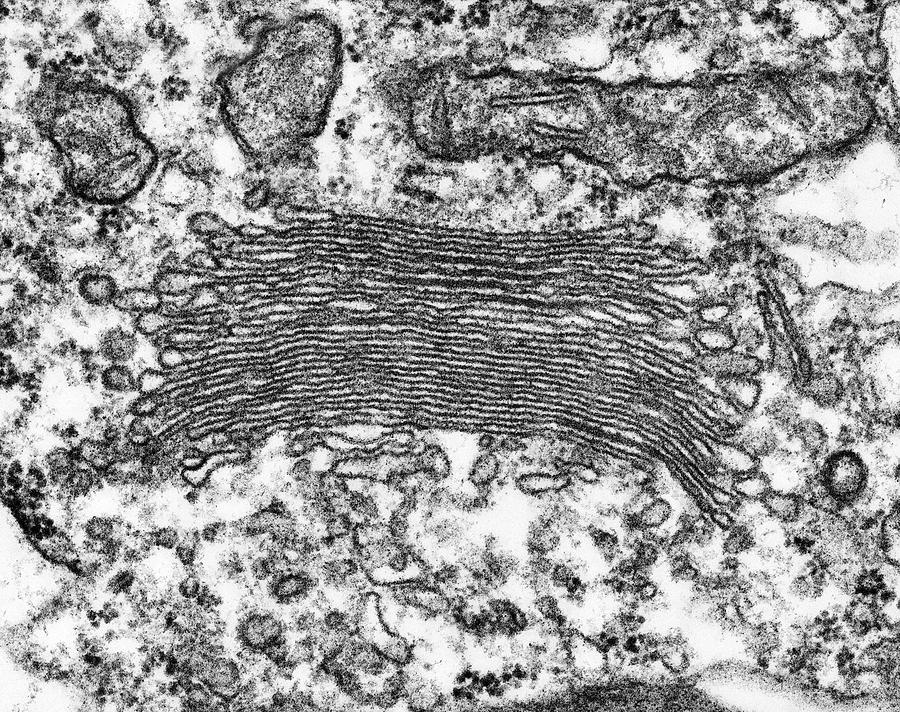This is a horizontal, rectangular black-and-white image, reminiscent of something you might see under a microscope or perhaps an abstract design by an artist. The background is predominantly white, scattered with various shapes and densities in shades of gray and black, creating a grainy texture. Prominent in the center are numerous parallel lines, which are not strictly straight but have rounded ends, resembling elongated strands or strings with hoops at each end. These central lines give the impression of striations or strung-together segments, much like lines viewed through a cellular lens. Above this central region, there are three large sections bordered by thick black lines, each containing an assortment of shapes. The upper left hosts two large blob-like shapes, while the upper right features a longer, oval-shaped figure that could be likened to a giant worm. Scattered across the image are various shapes, including completely round, filled-in circles, oblong dark gray forms, and tiny clusters of black and gray dots. The composition as a whole appears to be a mix of microscopic detail and artistic abstraction, with one clear spot punctuating the complex design.